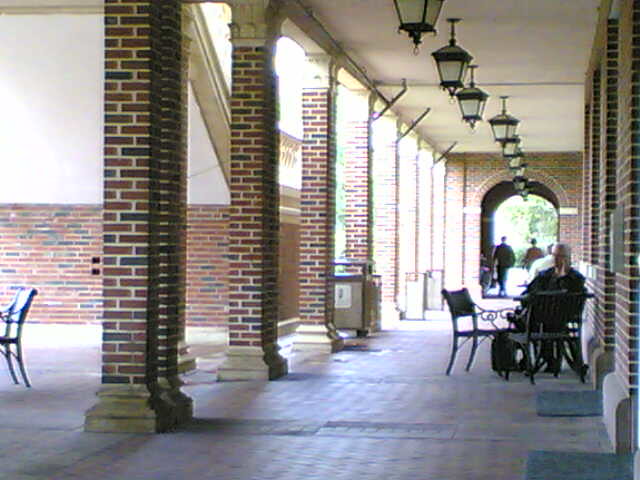This horizontal, full-color photograph captures an outdoor passageway adjacent to a large, brick building, possibly part of a college campus. The scene is bathed in sunlight, highlighting the extensive brickwork that features both lighter and darker shades. On the left side, brick pillars line the passageway, with a secondary building in the background that has brick at the base and stucco above. Tables with chairs are interspersed along the area, including one occupied by an older gentleman in the lower left corner; he appears to be sitting at a black table, possibly using his phone. Another chair stands alone to the far left. Above, black lantern-style lights hang from the overhead ceiling, adding a touch of classic charm to the setting. In the distant background, an archway framed in brick draws the eye, and two or three people can be seen walking away from the camera. Additional details include a garbage can near the left side and the sense of a bustling yet serene environment.